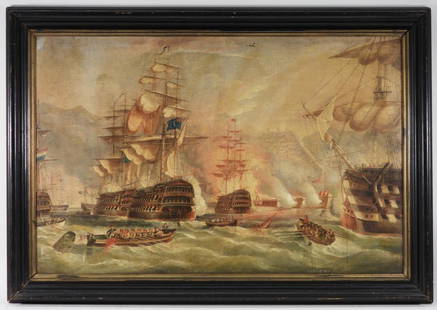The image depicts a historic oil painting encased in a dark wood frame with intricate carvings, set against a white background. The scene captures a dramatic naval battle, likely from the 16th or 17th century, fought on a tumultuous, white-capped sea. Central to the painting is a large, three-storied ship with four tall masts, their white sails billowing as it leans slightly to the right. This vessel is juxtaposed with several smaller boats manned by oarsmen, furiously paddling through the rough waters. In the hazy distance, another tall ship emerges through a smoky horizon, shrouded in the chaos of battle. The sky above is filled with swirling clouds and smoke, punctuated by hints of blue, suggesting the relentless cannon fire and the clashing of ships. The overall scene emanates a sense of ferocity and movement, capturing the intensity of the maritime conflict.